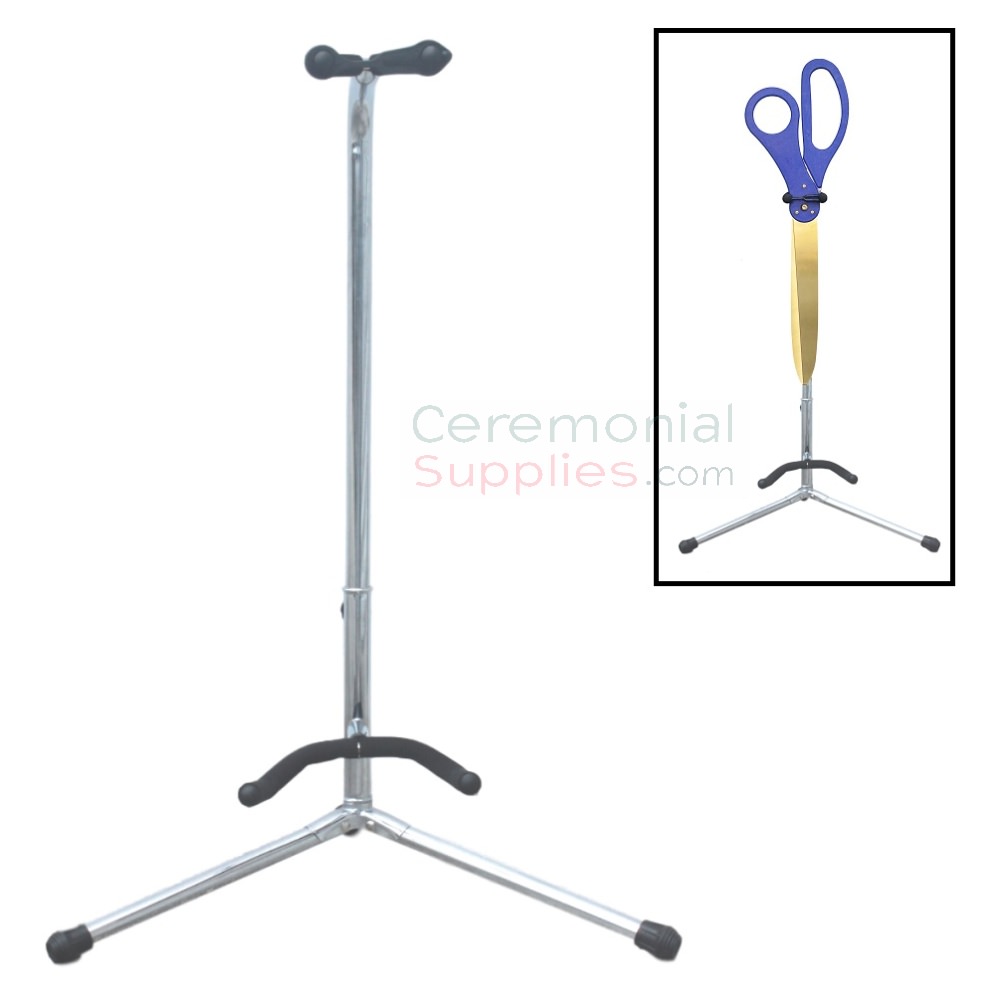The image depicts a metal tripod stand designed to hold scissors, characterized by its silver construction and various black rubber components for stability and grip. At the base, two visible legs spread outwards with rubber tips, accompanied by a small half-arc bar joining them. The stand might have a third leg at the back, obscured from view. Black rubber grips, resembling close-set bike handles, are positioned near the top. On the right side of the image, a rectangular framed picture showcases a similar stand holding a pair of blue-handled scissors with gold cutters. The photograph prominently features the text "ceremonialsupplies.com" in the center, indicating the intended use of the stand as a ceremonial scissor holder.